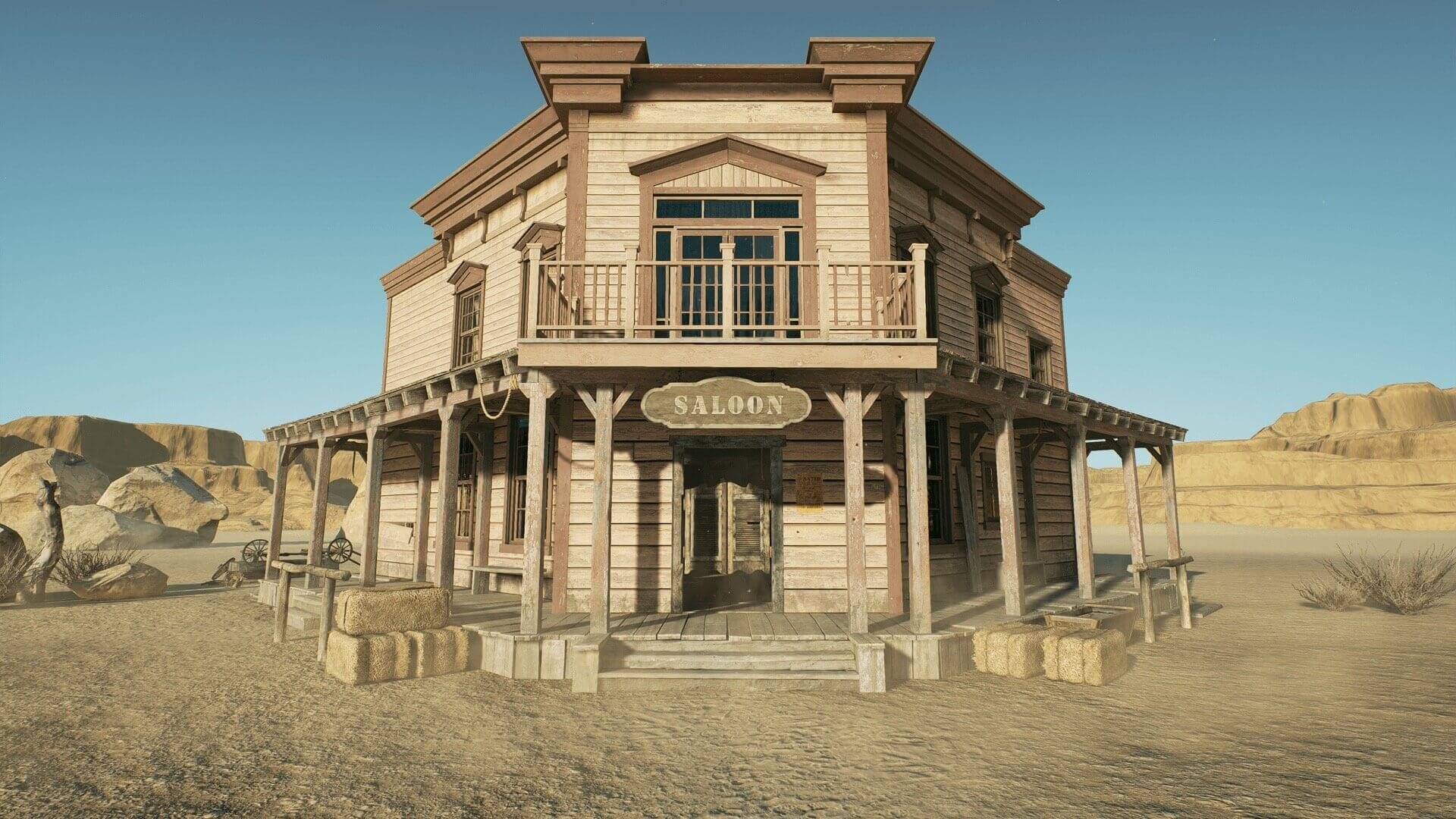In this photorealistic image of a Wild West saloon, depicted in the center of a desert setting, the saloon building conveys a sense of the late 19th century. The structure is predominantly constructed of wood with shades of gray, tan, beige, and darker brown tones that highlight the age and weathering of the facade. A sign proudly hangs above the entrance, reading "Saloon," marking its purpose unmistakably. The saloon features a large, wraparound open-air porch supported by columns, with bales of hay flanking the entrance, hinting at a place where horses could be tied up. The iconic swinging double doors are wide open, inviting glimpse into its rustic interior. The second floor boasts a balcony, suggesting rooms for guests above. The ground surrounding the building is bare dirt, void of vegetation, emphasizing the harsh desert environment. In the backdrop, sandy mountains and rocky terrain under a sky that transitions from light blue to dark blue provide a stunning contrast to the saloon’s earthy tones. No other buildings are in sight, amplifying the saloon’s isolation in this professional, unpainted, and non-AI-generated photograph.